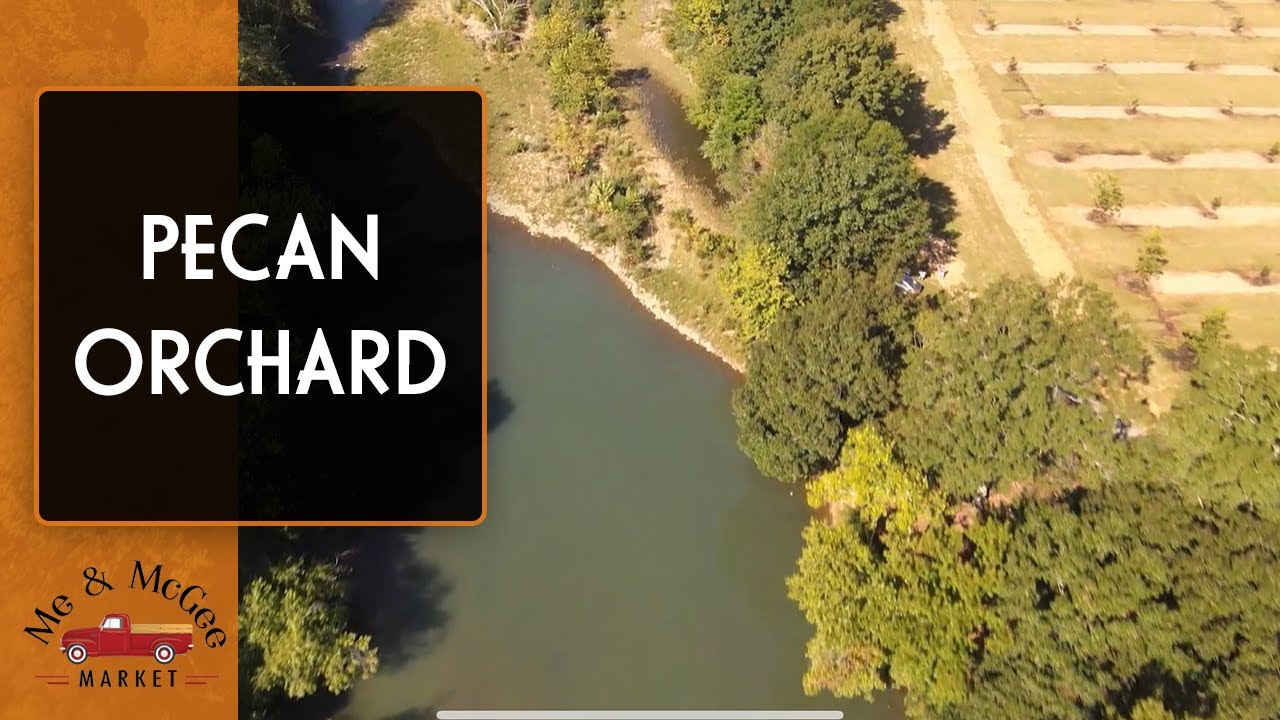This captivating aerial photograph showcases a serene landscape where a muddy, greenish-brown river flows on the left side, bordered by lush, vibrant trees. Above these trees, a dirt road stretches across a verdant but slightly faded field to the right. Adjacent to the road, rows of trees are separated by light-colored soil, and green grass fills the spaces between the rows. The trees near the river appear greener in contrast to the grass. On the left side of the image, a prominent black box displays the text "Pecan Orchard" in white letters, beneath an orange label with white lettering that reads "Me and McGee Market," and a red pickup truck can be seen underneath this arched signage. The scene is a beautiful depiction of the rural peach orchard associated with Me and McGee Market.